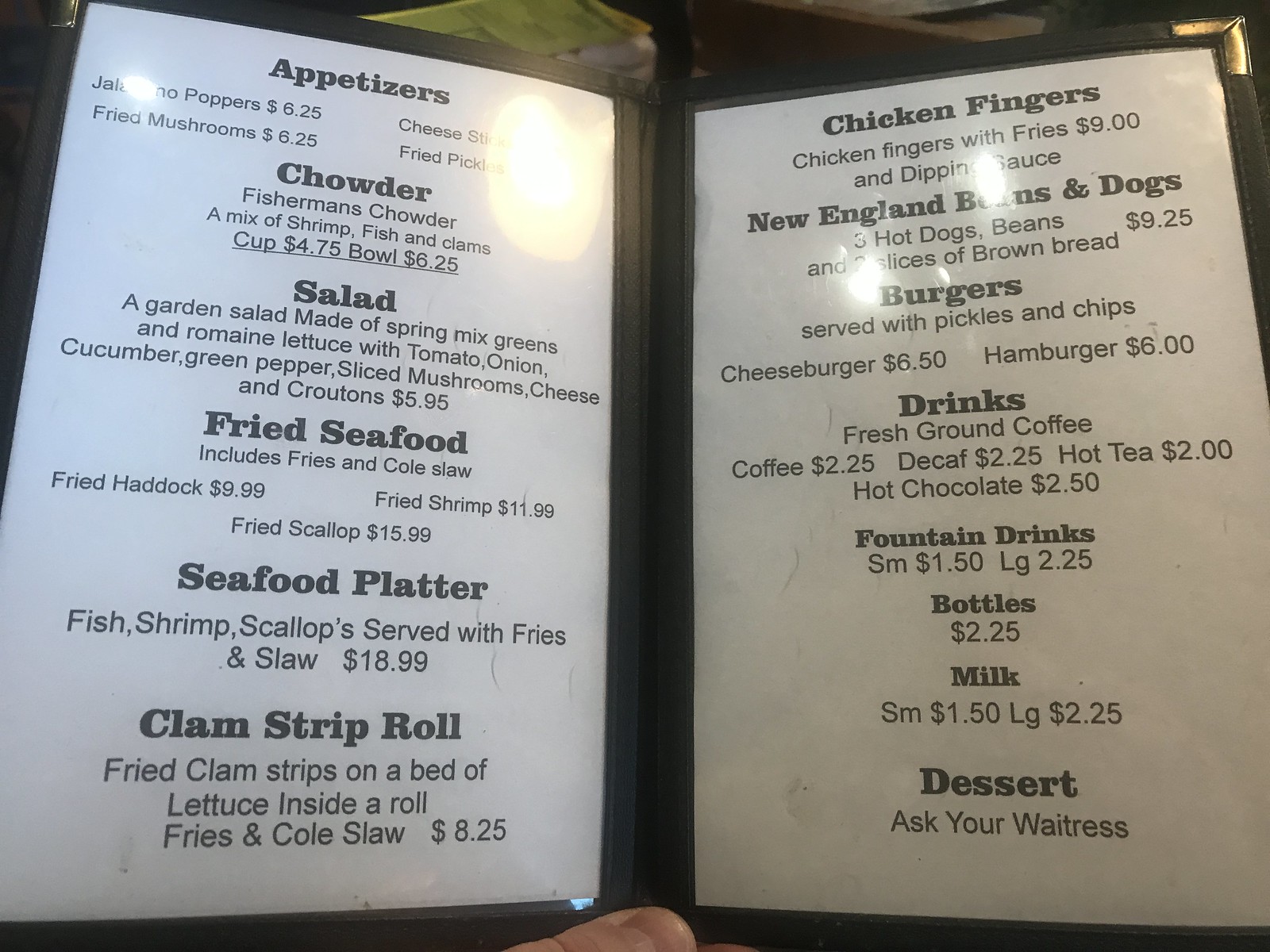In the image, we see an open menu held up by someone's thumb at the bottom, suggesting the person is reading it. There is noticeable glare on the menu pages, indicating an overhead light source. The menu is spread across two pages; the background of each page is white with black text, and the corner of the right page has gold edging.

On the left page, the sections listed are appetizers, chowder, salad, fried seafood, seafood platter, and clam strip roll. Each item has a brief description in a lighter, less bold font beneath the main titles, accompanied by the prices.

On the right page, the menu continues with sections for chicken fingers, New England beans and dogs, burgers, drinks (including fountain drinks, bottles, and milk), and dessert. The titles are in a bold black font, while the descriptions and prices are in a lighter black font. Notably, the dessert section instructs patrons to "ask your waitress," with no specific items or prices listed, unlike the other sections that provide descriptions and pricing or just pricing in the case of the drinks.